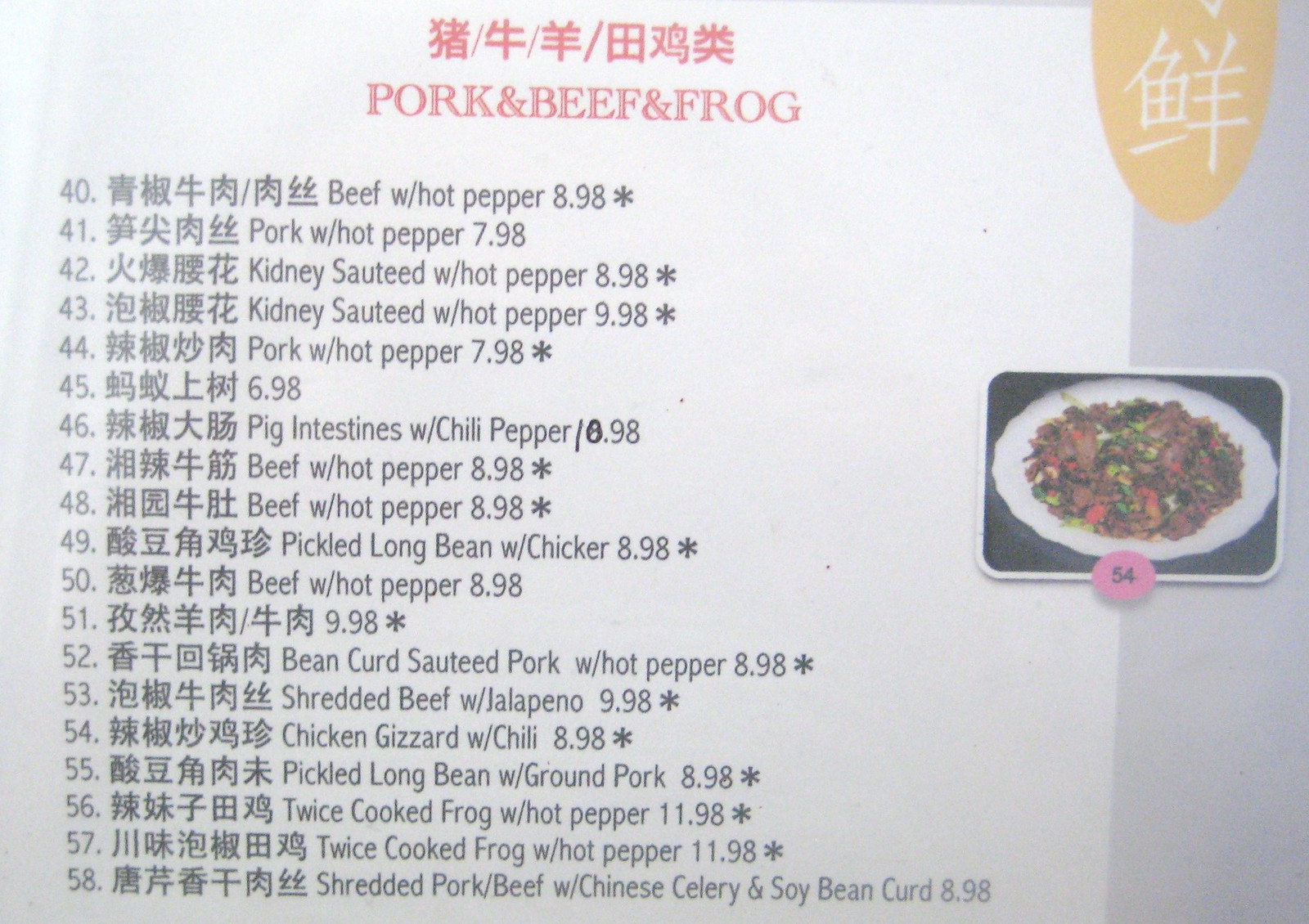Close-up image of an Asian restaurant menu featuring items in both Asian characters and English. Starting from the top, there is a row of Asian characters, followed by English translations listing items such as "Pork," "Beef," and "Frog." On the left side, the menu items are numerically organized, starting from number 40 and descending to number 58. Each row begins with Asian characters, followed by the English item name and the price, with approximately 15 items in total.

In the upper right corner, a yellow oval icon with white Asian letters is visible. Near the center-right edge, a rectangular image displays a plate of food labeled with a purple dot reading "54." According to the menu, item 54 is "Chicken Gizzard with Chili," priced at $8.98, denoted with an asterisk. The background of the image is predominantly white, transitioning to gray on the right side. This meticulous menu layout, characteristic of a Korean or Chinese restaurant, is captured with exceptional clarity.